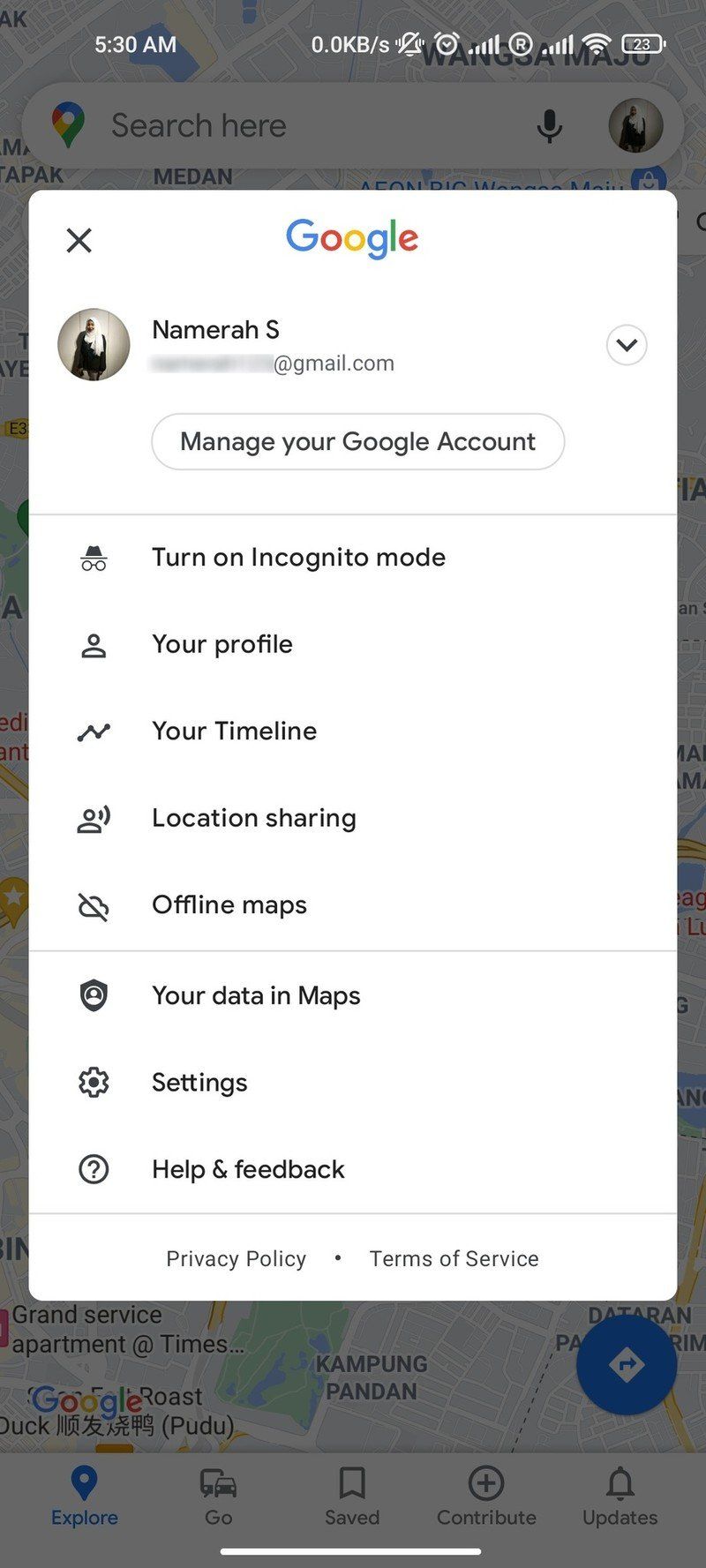The image is a screen capture taken from a mobile device. The screen's background displays a grayed-out map, which appears muted and partially obscured. In the upper-left corner of the screen, the time is clearly visible, indicating 5:30 a.m. Below the time, there is a prominent, white, rectangular window with rounded corners. 

At the top of this window, the colorful Google logo is prominently displayed. Directly beneath the logo, a black-and-white profile image of a person is shown within a circular frame, alongside the profile name "Na Mera S" written in black text. 

Below the profile section, there is a button labeled "Manage your Google Account," inviting the user to access account settings. Further down, a list of Google-related options is presented, including "Turn on Incognito mode," "Your profile," "Your timeline," "Location sharing," and "Offline maps."

This detailed layout showcases various functionalities and account management options within the Google interface on a mobile device.